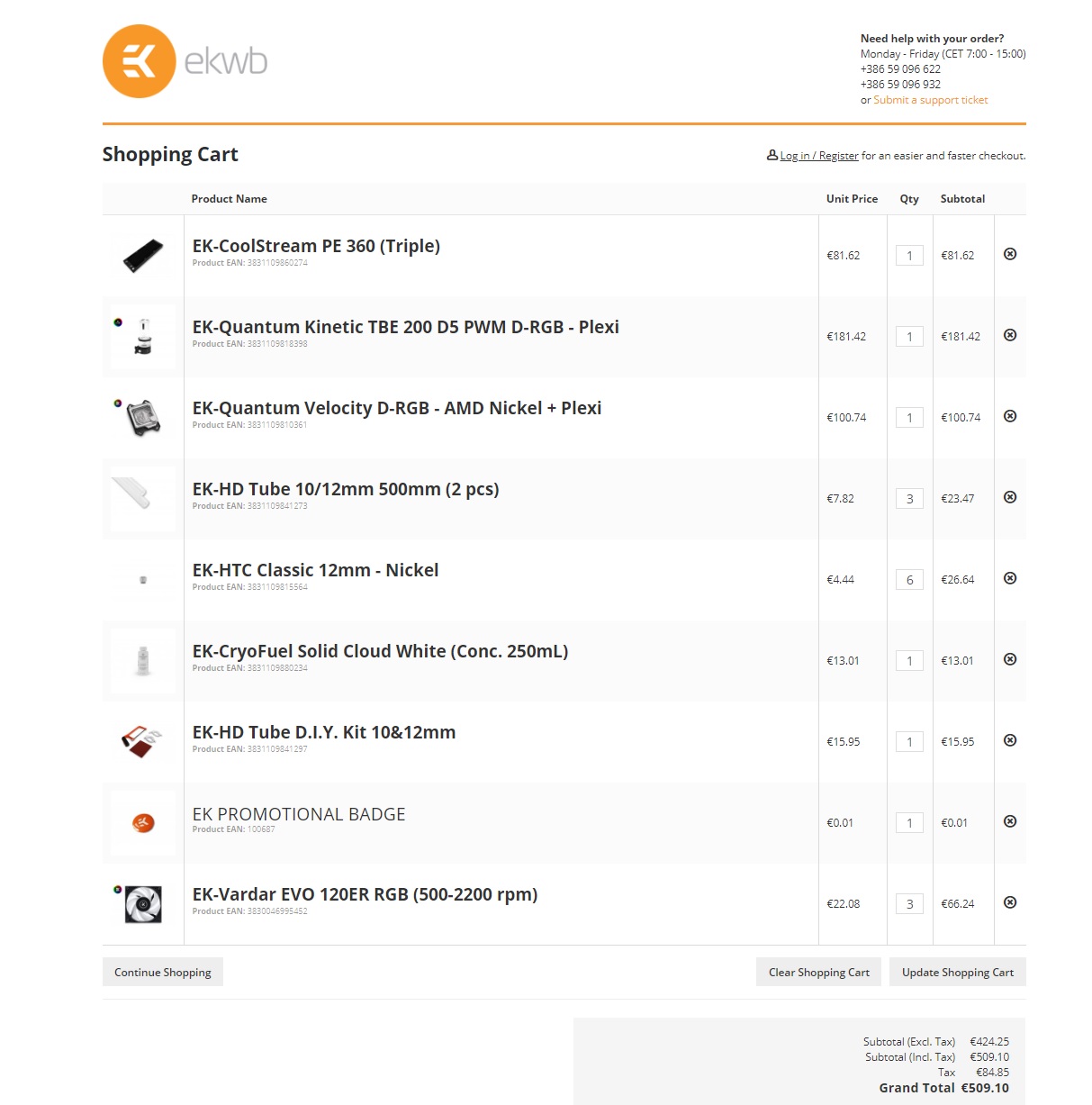This image captures a detailed screenshot of an online shopping cart webpage. The top section features a header with a sleek, minimalist design set against a white background. On the left side of the header, an orange logo with a distinct symbol is prominently displayed next to the brand name "ekwb" in lowercase letters. Moving rightward within the header, contact information including a phone number and business hours is listed, accompanied by an option to submit a support ticket. This header section is neatly separated by a horizontal yellow-orange line that spans the entire width of the page.

In the main body of the webpage, the top left corner prominently displays the text "Shopping Cart." Directly below, an organized layout showcases the items added to the cart. Each row is dedicated to a different product and includes a small image of the product, the product name, the unit price, the selected quantity, and the subtotal for that particular product.

Towards the bottom of the page on the left, a button labeled "Continue Shopping" invites users to add more items to their cart. On the opposite side, two buttons labeled "Clear Shopping Cart" and "Update Shopping Cart," both in gray, offer options to either empty the cart or update the quantities of the selected items.

At the very bottom of the page, a gray box summarizes the financial details of the cart. This box itemizes the subtotal excluding tax, subtotal including tax, the tax amount, and the grand total. Each financial figure is aligned to the right for easy readability.